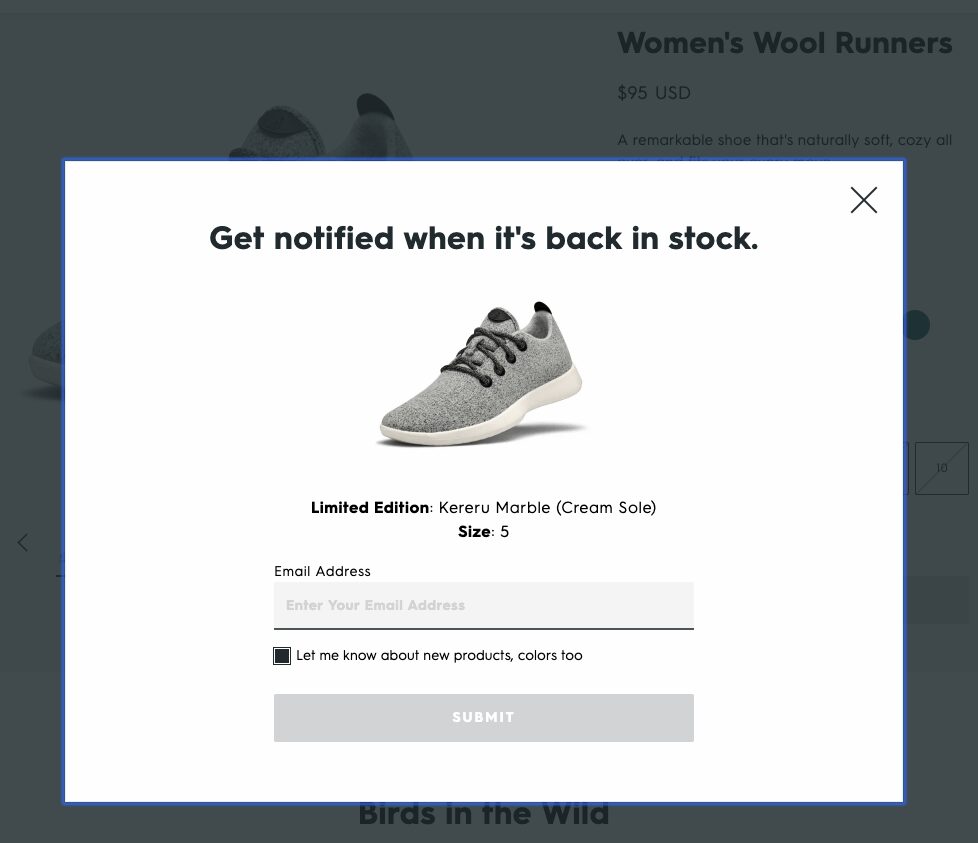The image, captured from a website page, prominently displays the text "Women's Wool Runners" in the background, indicating the type of product being showcased. Featured on the page are several pairs of shoes, which are the focus of the display. Overlaid on the background is a white pop-up that somewhat obscures the underlying webpage. This pop-up contains a message stating "Get notified when it's back in stock" with an 'X' icon in the upper right corner for closing the notification. 

Within the pop-up, there's a detailed product description which reads: "Limited Edition Kara Rue Marble Cream Sole" alongside a specification that the shoes shown are in size 5. Below this information is a field prompting the user to enter their email address, accompanied by an optional checkbox labeled "Let me know about new products, colors too." At the bottom of the pop-up is a gray submit button with the word "Submit" in white, indicating its functionality, which will become active after an email address is entered and the checkbox is selected.